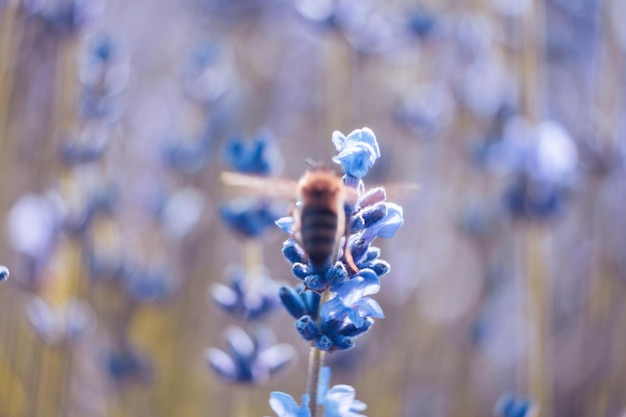The photograph captures a vibrant scene where a bumblebee, with its gold and brown striped abdomen, is in motion, hovering over a blue-purple flower. The bee's wings are extended out to the sides, appearing almost T-shaped due to the motion blur. Surrounding this main flower are more clusters of the same blue-purple flowers, forming long, cylindrical shapes on brown, slender stems. The flower in the foreground sharply stands out with its delicate petals, contrasting against the background flowers, which fade into a gentle blur. The overall composition beautifully freezes the moment of the bee collecting nectar amidst this sea of colorful flora.